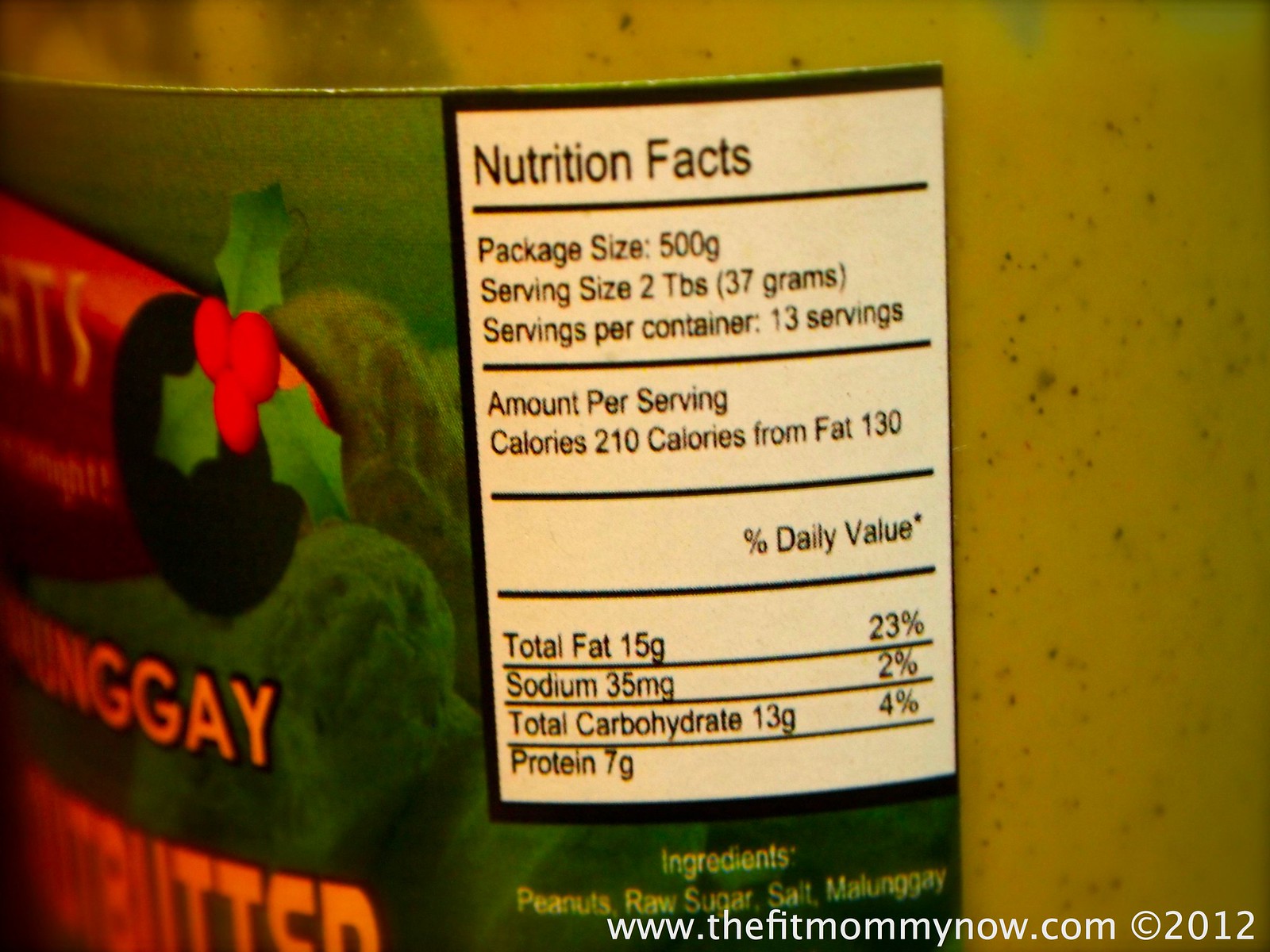The image captures an up-close photograph of a nutritional facts label on a round glass jar containing a creamy, light greenish-yellow substance with black specks. The label features a prominent green and red color scheme, with the red text bordered in black. Partially visible text on the label includes "GGAY" and "B-U-T-T-E," suggesting it may be a type of nut butter. In addition to the nutrition facts, which are displayed within a white rectangle in the center of the image, the label provides details such as package size (500 grams), serving size (2 tablespoons or 37 grams), and servings per container (13). The caloric information is listed, with each serving containing 210 calories (130 calories from fat). The nutritional breakdown includes 15 grams of total fat (23% DV), 35 milligrams of sodium (2% DV), 13 grams of total carbohydrates (4% DV), and 7 grams of protein. Ingredients listed are peanuts, raw sugar, salt, and malunggay. At the bottom of the image is a watermark that reads "www.thefitmommynow.com, copyright 2012" in white text.